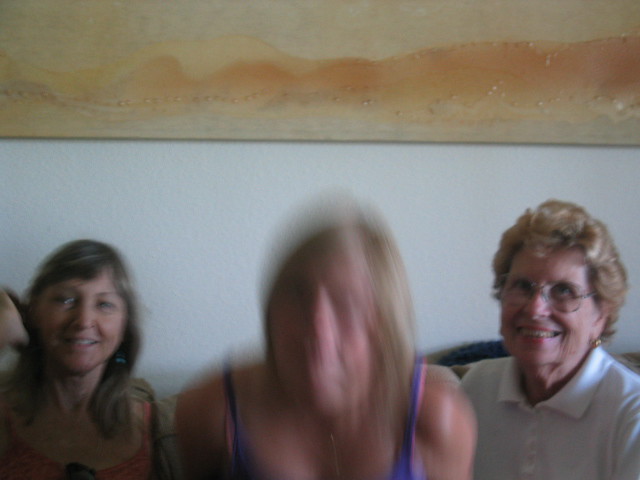In this photograph, three white women are seated together in a cozy home setting, capturing what appears to be a cherished family moment. The middle woman, caught in motion, is slightly blurred due to the long shutter speed, while the other two women on either side are more in focus, though the focus remains soft overall. The woman on the right, who appears to be the eldest, radiates warmth with her gentle smile. The woman on the left, younger than the one on the right, also beams at the camera. The backdrop features the lower portion of a vibrant piece of modern art that extends across the frame, adding a splash of color and contemporary flair to the scene. Their expressions and the intimate setting suggest a heartfelt family gathering.